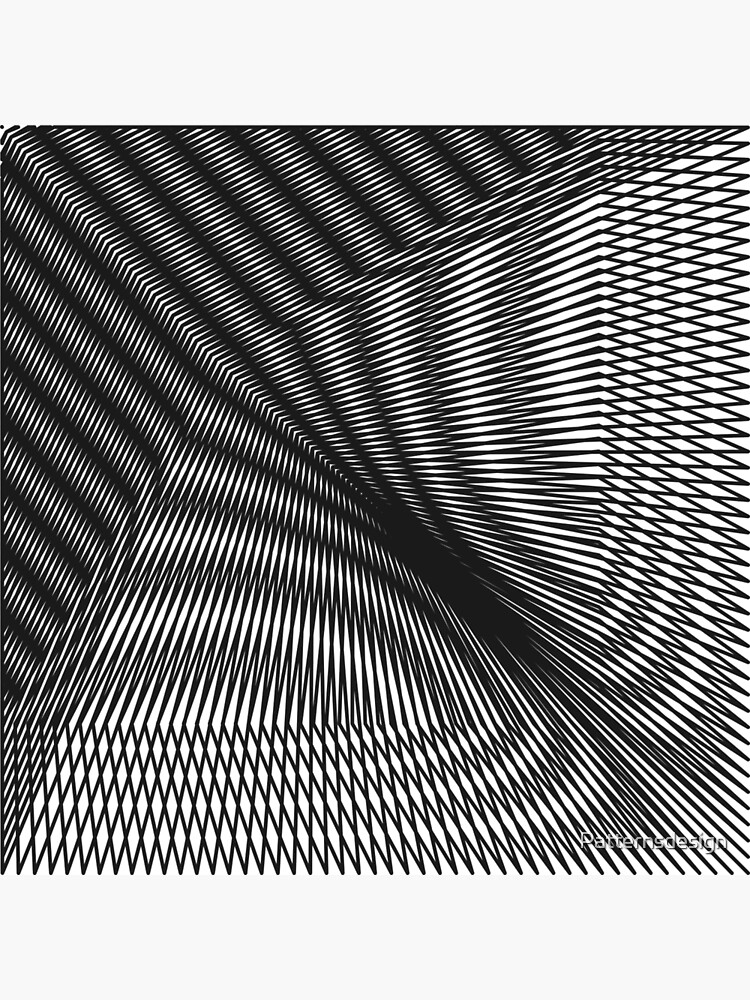This digital image features a complex black and white geometric optical illusion designed to play tricks on the eyes. The upper left corner showcases grey spiral lines against a black background, creating a dynamic visual effect. As the lines progress diagonally downwards, they transition and diverge, with some continuing straight down or horizontally to the right. This shift in direction segments the image into various patterns, including black and white diamonds and triangles, which appear to become larger towards the bottom right where text reads "patterns design." The illusion creates a sense of depth, reminiscent of a 3D metallic gate or a tunnel, thanks to the intricate interplay of shapes and shading. The entire composition, devoid of any color, masterfully manipulates perception, making it seem both flat and deep simultaneously.